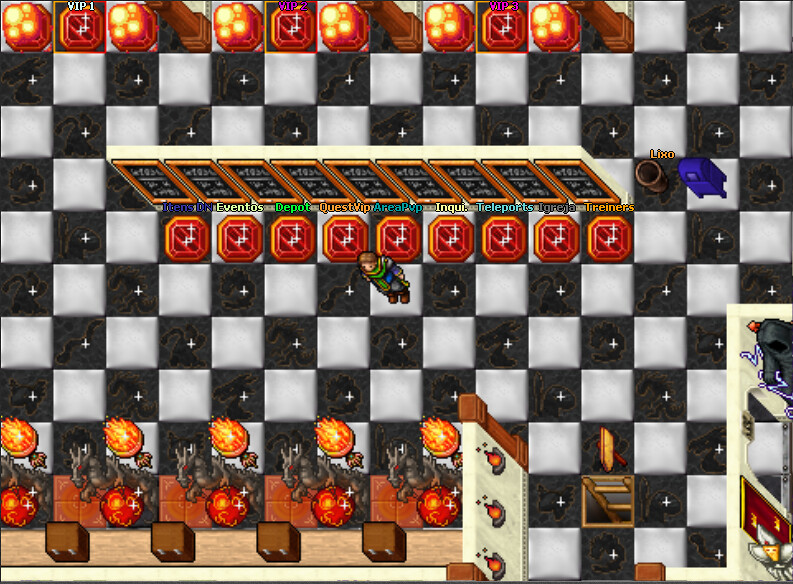The image depicts a highly-detailed pixel art-style video game screenshot, likely from a PC game. Dominating the view is a black and white checkerboard floor intricately intermixed with white crosses. The checkerboard is punctuated by conspicuous, glowing ruby-red emblems arrayed in the center, each bearing labels such as "Eventos," "Depot," "Quest VIP," and "Area PVP," suggesting multiplayer elements.

At the top margin, several squares feature a dynamic mix of glowing orange and magenta orbs and brown columns, which complement the ruby emblems laid out in front of black rectangles with brown borders that resemble chalkboards with white text. The bottom of the image is adorned with decorative dragon statues, some of which are surrounded by intricate fire-like ornaments, adding to the game's thematic richness.

In the very center stands a character, potentially the main protagonist of the game, further emphasizing the interactive and immersive nature of the in-game environment. The scene exudes a nostalgic 8-bit aesthetic, rich with vibrant colors and detailed designs that hint at an intricate game board or maze-like structure, enticing the player to explore.